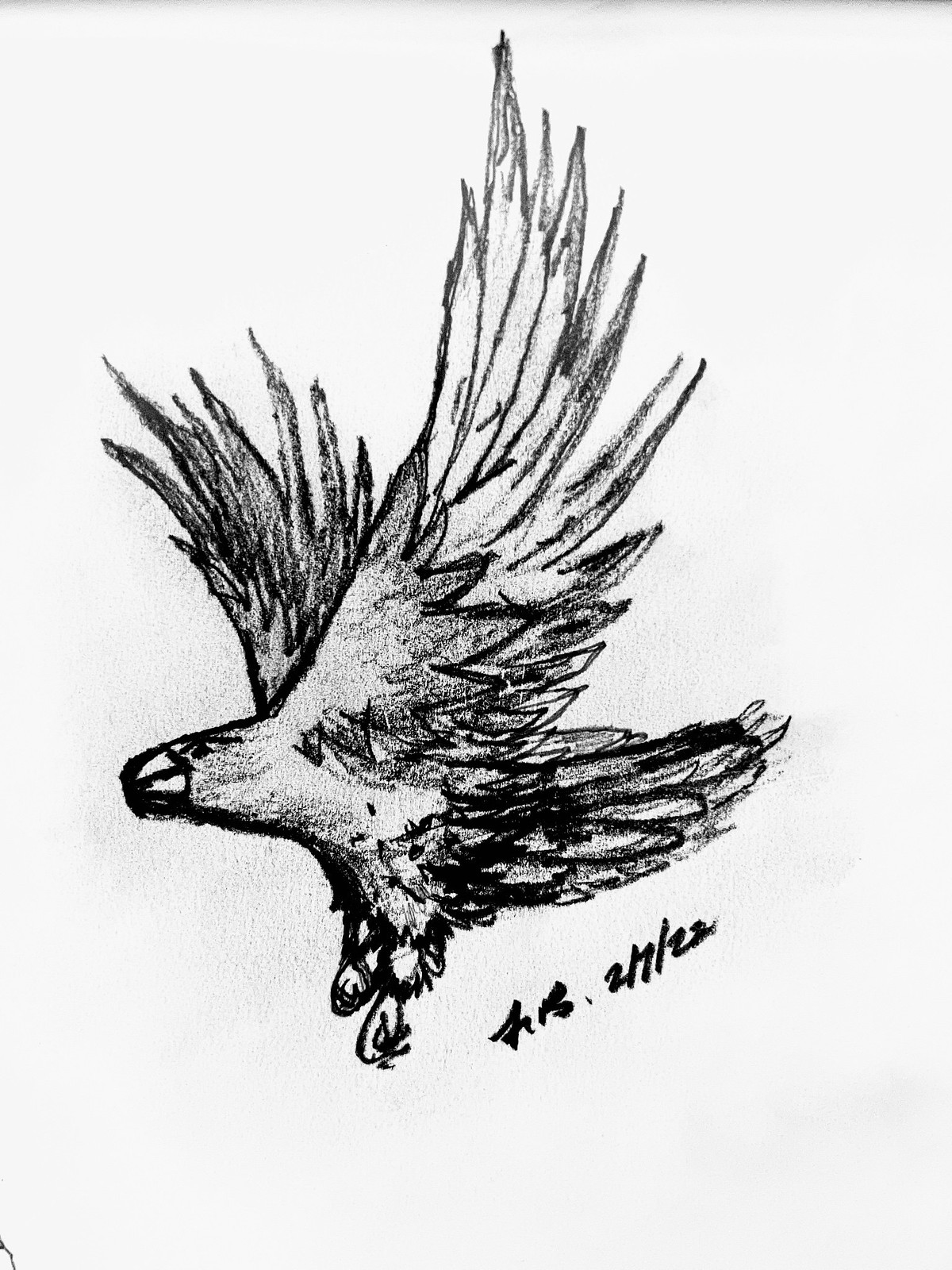This image features a pencil or charcoal-style sketch of an eagle in flight on white paper, marked by the date 2-7-22 and a signature that appears to be "FB." The eagle, depicted in black and white with heavy line work, showcases a combination of shadow and shading, particularly on its wings and tail feathers. Its wings are spread wide and upward in a V-shape, ending in pointed tips, while its talons hang prominently below. The bird’s head, with a small hooked beak and relaxed eyes, faces towards the left. The shading on the wings and tail feathers adds depth, although some areas appear smudged. The overall composition has a minimalistic background, focusing solely on the detailed representation of the eagle in mid-flight.